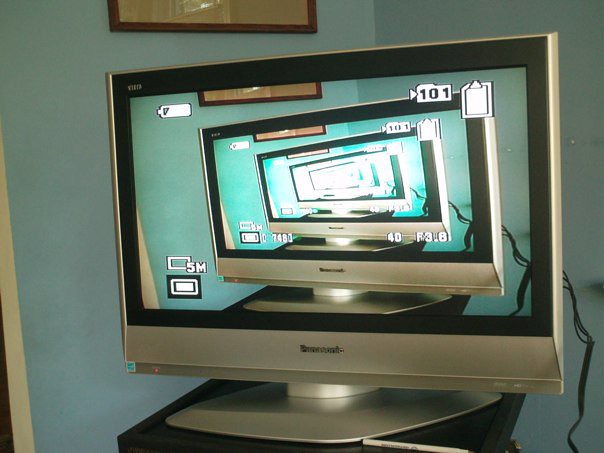This photograph captures an older silver-framed LCD computer monitor with a black border, sitting on a black desk with a diamond-shaped base. The backdrop consists of light blue walls, and a brown-framed picture with a tan background is visible hanging above the monitor. The monitor's screen displays an infinity effect, showcasing a recursive image of itself that appears smaller and smaller, repeating approximately five times into the distance. This creates a visually striking "image within an image" effect reminiscent of the concept of inception.

Additional details on the monitor's display include a battery indicator, a "5M" label in the bottom left corner, and "101" within a rectangular box in the upper right corner, resembling photographic or emoji-like settings. Visible wires extend from the back of the monitor, trailing off to the right side both in the actual scene and within the repeated images. A pen is noted to be resting on the desk near the monitor. The meticulous setup and recursive image create an engaging visual narrative that transcends the simple setting.